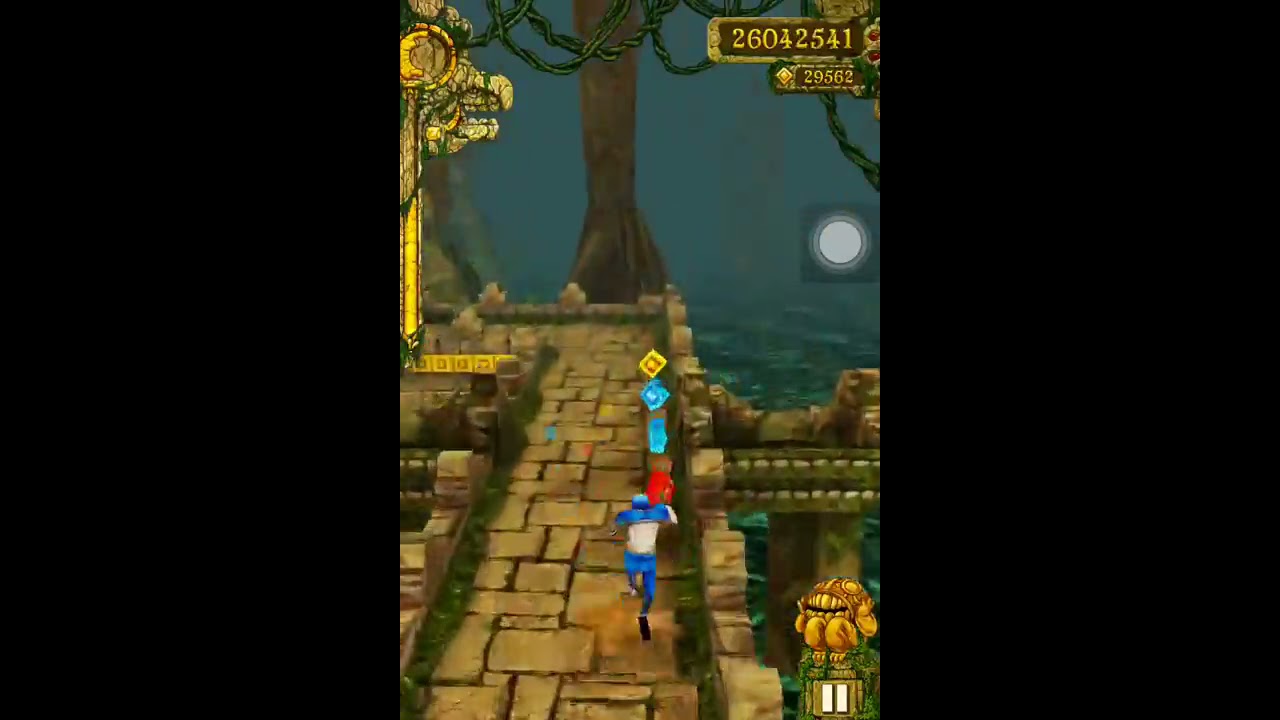This image appears to be a screenshot from a mobile endless runner video game, featuring a character dressed in blue. The character is seen running down a brick or stone path from a behind-and-over vantage point, oriented centrally towards the bottom of the vertical display, which suggests it is optimized for a mobile screen. Surrounding the path, there is lush greenery, including vines and foliage, suggestive of a jungle environment that features stylistic elements reminiscent of South American, specifically Aztec or Mayan, stone structures. 

Rotating crystals in blue, gold, and yellow hues are positioned before the character, indicating obstacles or collectible items in the game. In the scene's mid-ground, there is a noticeable large tree trunk, further enforcing the jungle setting, with some green ropes loosely hanging at the top of the image. A body of greenish water is visible to the right of the path, adding more detail to the environment.

The upper left corner of the image displays textual numerical information, specifically "260-42541" with "29562" beneath it, implying some form of score or in-game statistic. Along the right and left sides of the screen, an interface element resembling a reticle or keypad is visible, likely part of the game's control scheme. The prevalent colors in the image include red, yellow, aqua blue, regular blue, gold, beige, brown, grayish blue, black, white, gray, and dark green, demonstrating a rich and varied color palette typical of digital video game art styles.